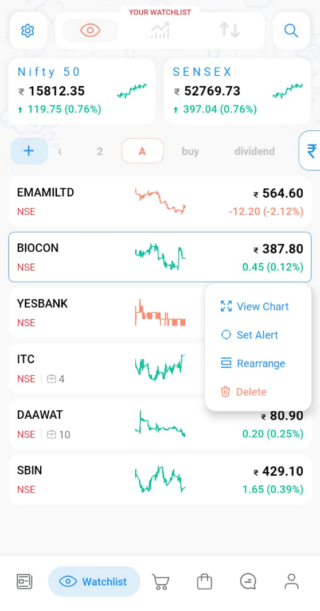The image displays a comprehensive layout of a stock market watch app. At the top, the title "Your Watch List" is prominently highlighted in red, with a settings button and an eye icon positioned just below it. Beneath this, there are several interactive elements including a bar graph icon with intricate lines, and arrows indicating upward and downward trends, all encapsulated within a single rectangular box.

Adjacent to this box, there is a search button that allows users to look up specific stocks. Below the search bar, notable market indices "Nifty 50" (spelled out in capital letters "N-I-F-T-Y 5-0") and "Sensex" (with emphasis on "SE" and "SEX") are featured, displaying their respective pricing details.

Further down, the interface includes a plus button, an "A" button for text modifications, a buy button for stock purchases, and a dividend button for viewing dividend information.

The main section of the interface lists various stocks, each accompanied by a miniature chart indicating price trends and the actual stock price. For example, the first stock listed is "EMAMI LTD," depicted with a downward trending chart and a price of 564.64 yen.